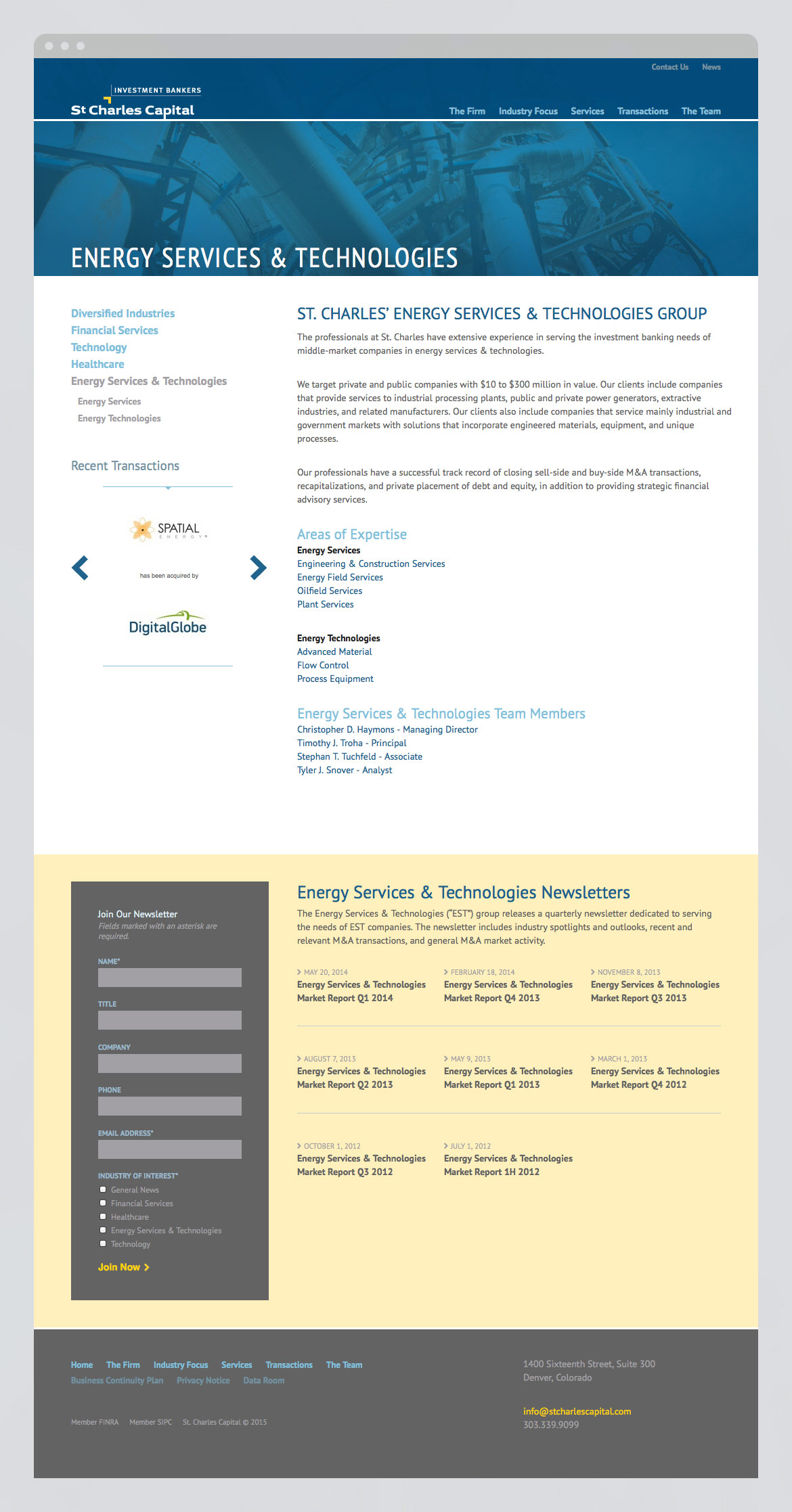This image showcases a professional-looking webpage designed with a sophisticated palette of white, dark blue, dark gray, light gray, and bright blue accents. The outer border of the page features a light gray background. At the top, a dark blue header spans the width of the page, prominently displaying a white logo in the upper left-hand corner that reads "St. Charles Capital" in bold white text, complemented by a small yellow flourish above the word "Charles." 

On the right-hand side of this header, there is light blue text with navigational links labeled "Affirm," "Industry Focus," "Services," "Transactions," and "The Team." In the uppermost right-hand corner, smaller gray text provides quick access to "Contact Us" and "News."

Below the header, an image featuring metallic scaffolding with a light blue overlay spans the width of the page. Overlaid on this image, in striking white text located at the bottom left corner, are the words "Energy Services and Technologies."

The main body of the webpage is introduced with a title in dark blue text stating "St. Charles Energy Services and Technologies Group." Beneath it, light blue text presents sections labeled "Areas of Expertise" and "Energy Services and Technologies Team Members."

On the left-hand side of the page, a vertical list of links in bright blue and gray offers navigation to various sections: "Diversified Industries," "Financial Services," "Technology," "Healthcare," "Energy Services and Technologies," "Energy Services," "Energy Technologies," and "Recent Transactions."

The footer is shaded dark gray and includes several important links in bright blue: "Home," "The Firm," "Industry Focus," "Services," "Transactions," "The Team," "Business Continuity Plan," "Privacy Notice," and "Data Room." To the right of these links, gray text provides a physical address: "1416th Street, Suite 300, Denver, Colorado," along with an email address in bright yellow: "info@stcharlescapital.com."